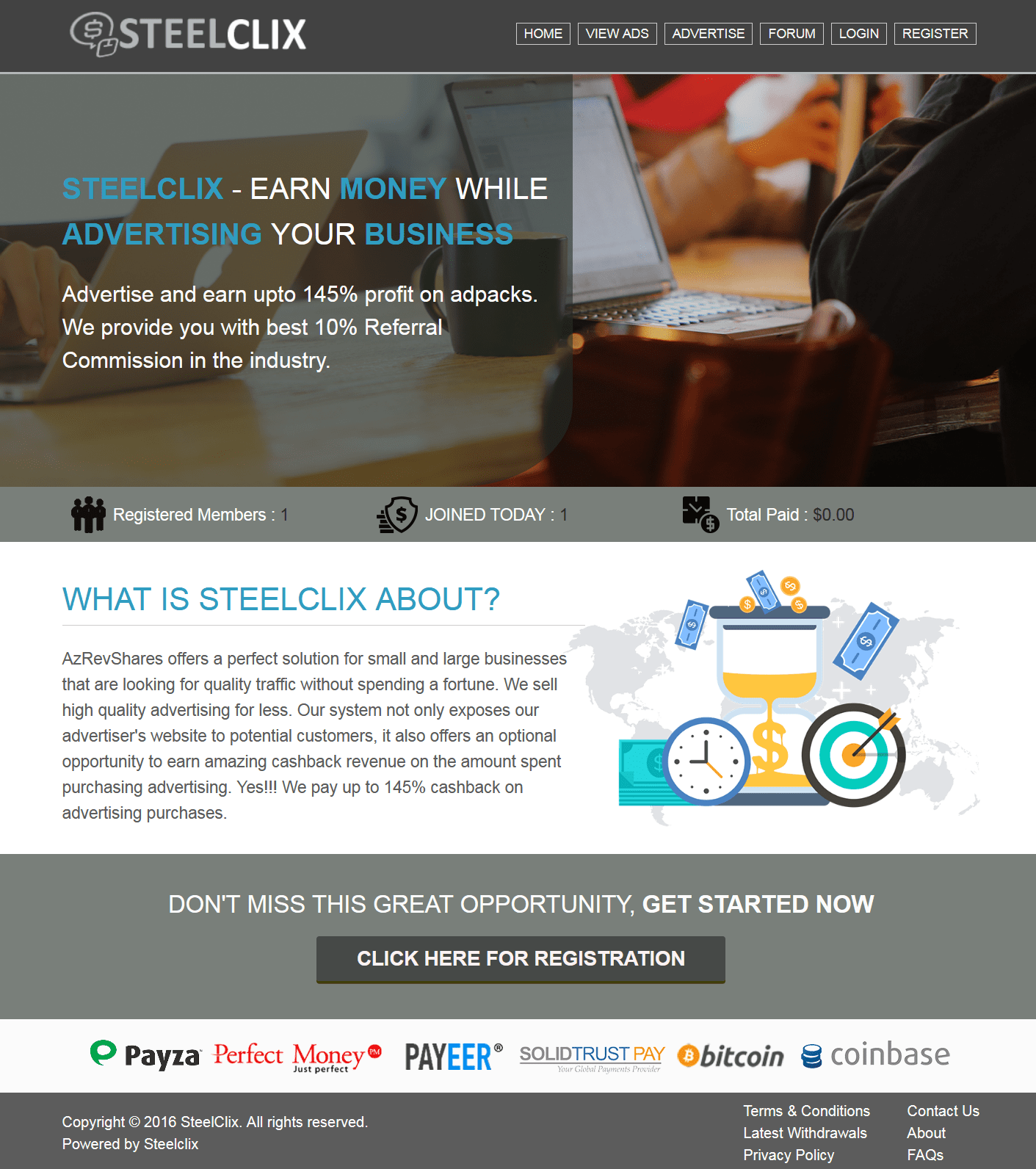In the image, the webpage titled "StillClicks" is displayed prominently in the top left corner. The top right of the webpage features navigation links labeled "Home," "View Ads," "Advertise," "Forum," "Login," and "Register." Dominating the left side of the main page is the slogan "StillClicks: Earn Money While Advertising Your Business," written in bold blue and white text. The tagline highlights potential earnings of up to 145% profit on ad perks and boasts a 10% referral commission—a standout in the industry. The webpage's background depicts a brown table with two laptops, two individuals' hands, and a black cup of coffee, creating a productive and business-oriented ambiance.

Directly below this, member statistics show "Registered Members: 1," "Joined Today: 1," and "Total Paid: 0," reflecting recent user activity. The center of the page features a blue heading titled "What is StillClicks About?" The description beneath, in black text on a white background, explains that StillClicks provides high-quality, affordable advertising solutions ideal for both small and large businesses. The site is designed not only to drive traffic to advertisers' websites but also to offer enticing cashback revenue of up to 145% on advertising purchases.

To the right of this section, there is a distinctive illustration of a yellow hourglass, a clock, a target symbol, and scattered coins and paper notes in blue, green, and yellow, symbolizing time, goals, and financial incentives. Below this, a call-to-action reads "Don't miss the great opportunity, get started now" with a button titled "Click Here for Registration," encouraging immediate engagement. Further down, payment options for the service are listed, including Payza, Perfect Money, Payeer, SolidTrustPay, Bitcoin, and Coinbase, offering a variety of methods for user convenience.